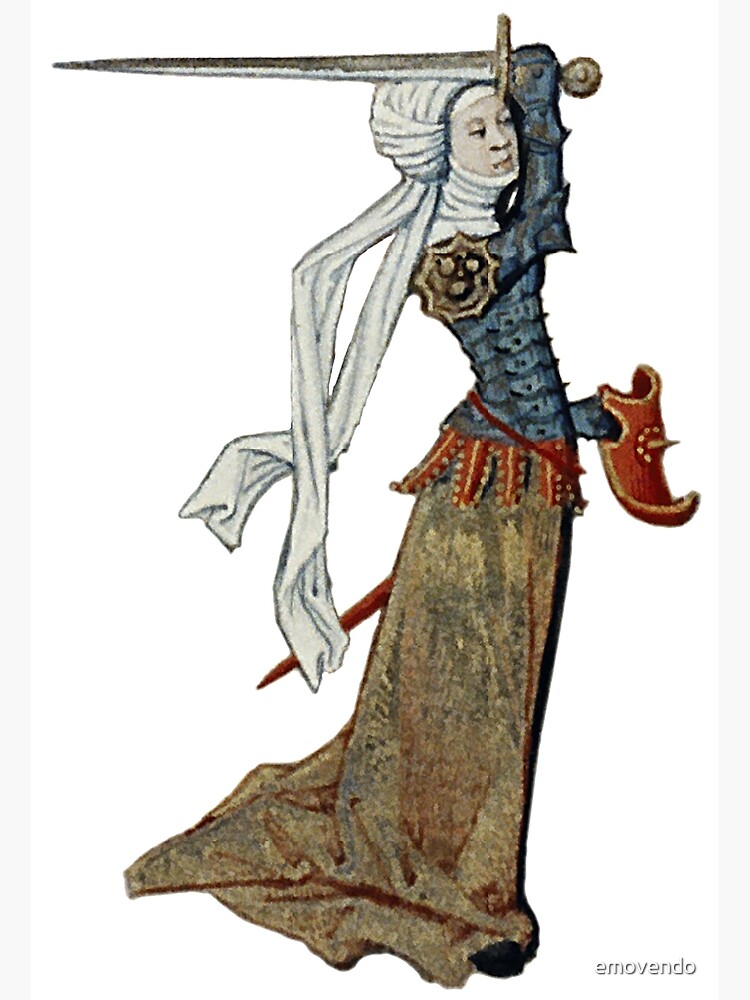The image is a detailed color print titled "Emovendo" located at the bottom right on a white background. It depicts a medieval woman with a very pale face, wielding a sword horizontally over her head, its tip pointing to the left. She wears a long, white, winding headscarf that covers her neck and hair, resembling a turban that flows down to the back of her brownish-colored long skirt, which extends past her feet, laying on the floor. Her attire includes a blue long-sleeved top made out of plated armor, featuring spurs or spiky armor on her shoulders. In her left hand, she holds a small red shield with a gold trim along the edges, while a brown, pointy stick—likely the sword's sheath—can be seen on the other side.